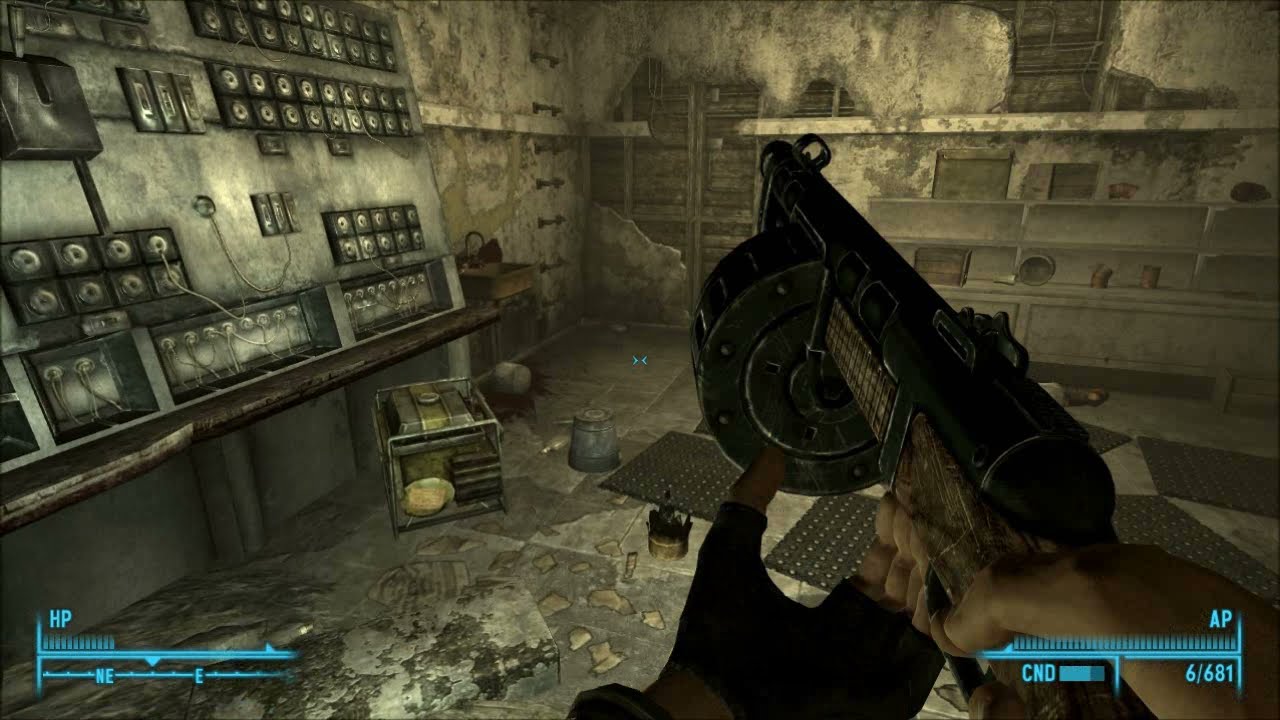The detailed caption for the image is as follows:

This is a high-definition, still frame from a first-person shooter video game, showcasing a dilapidated, industrial-themed room with advanced technological features. The room appears to be a power station with beige walls, one of which is damaged and contains a shelf or cabinet holding a box and a circular item on top. The right wall is equipped with numerous sockets. Emerging from the lower right corner of the frame are two human hands: the right hand grips a formidable black rifle while the left hand wears black, cut-out fingerless gloves. The interface includes light blue text at the bottom left and right corners of the screen, displaying gaming stats such as "HP," "E," "AP," "CND," and "64/681." The color palette of the image includes light blue, black, white, gray, dark green, olive, tan, brown, and gold.